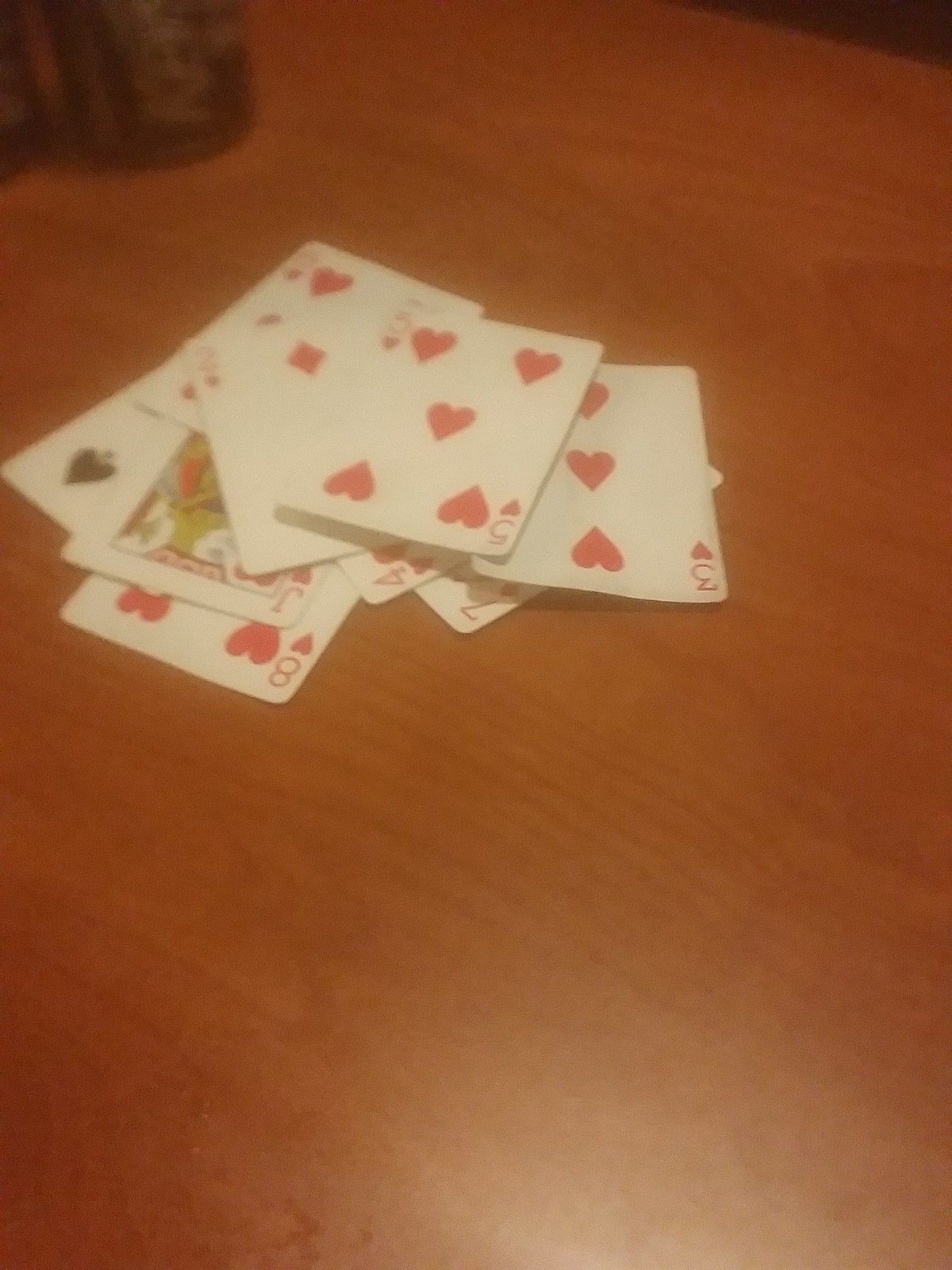This vertical, slightly blurry color photograph captures a wooden table with a collection of playing cards strewn across its surface. The rich brown wood, with its visible grain, subtly contrasts with the colorful array of cards, all facing up. The cards, haphazardly overlapping, include a 3, a 5, a 2, an 8, a Jack, a 4, a 6 of Hearts, a 7 of Diamonds, and a partially obscured Spade. Towards the back of the table sits an unidentified canister, possibly a drink or a candle, adding an element of curiosity. Light, perhaps from a window or an overhead source, gently illuminates the table, highlighting the cards and casting soft shadows. The background is predominantly dark, hinting at a dimly lit room with no discernible details or figures beyond the table and its contents.